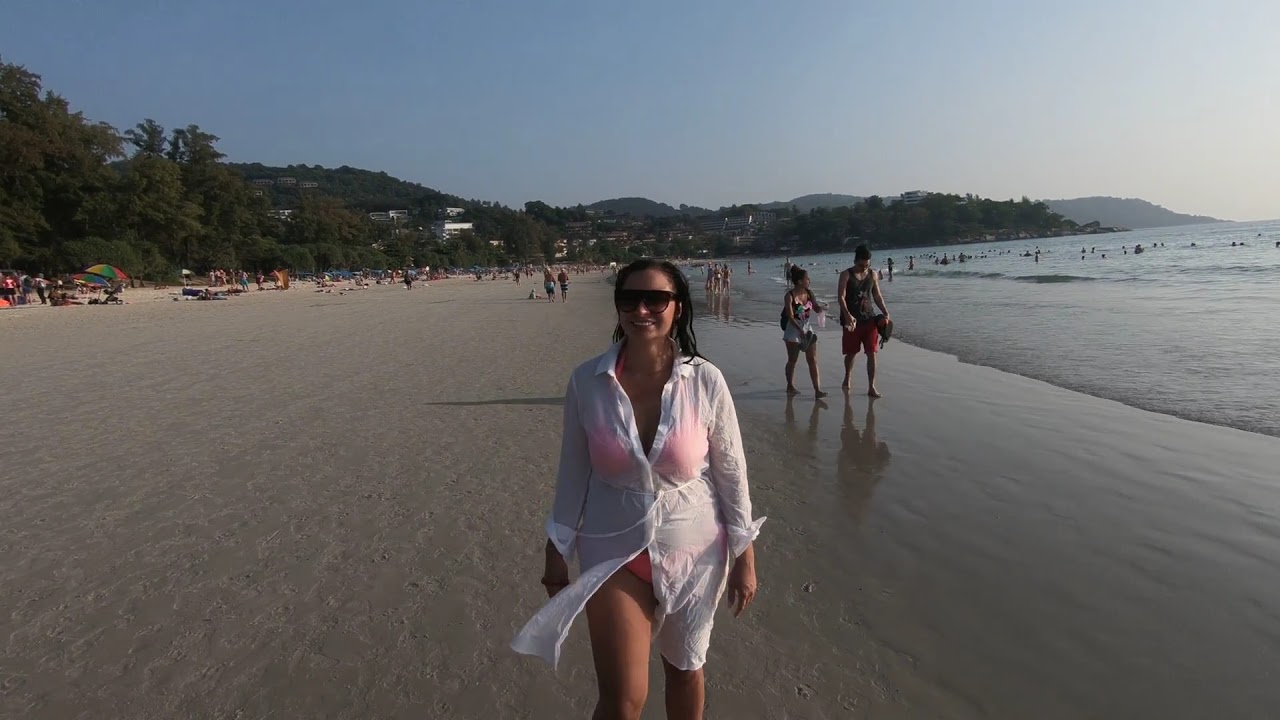The photograph captures a serene beach scene with a woman as the main focal point. She stands smiling and looking directly at the camera, her wet, shoulder-length black hair pulled back off her round face, and she wears very dark sunglasses. Clad in a sheer white shirt over a peach-colored bikini, she exudes a relaxed vibe. Behind her, the beach is sprinkled with people, some walking along the waterline and others lounging under umbrellas and on blankets. A couple, comprising a man in red shorts and a gray tank top, and a woman in light-colored shorts with a pink bikini top, strolls behind her. The gentle waves lap at the shore, and in the background, lush vegetated hills rise against the clear sky, adding to the idyllic ambiance.